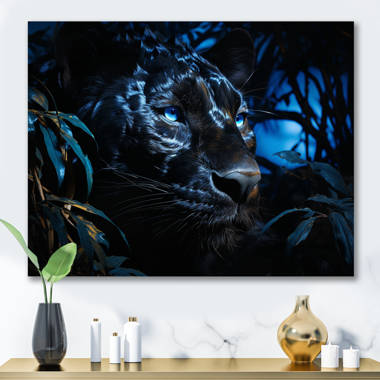This photograph captures a strikingly styled interior featuring a luminous gold shelf set against a white wall, accentuated by a dramatic piece of artwork above it. Hanging on the wall is a digital rendering of a close-up of a leopard, its intense blue eyes gleaming in the dark, shadowy forest, giving a black and blue tone to the image. Below the evocative artwork, the gold shelf, despite its wooden texture, shimmers as though metallic. On the left of the shelf, a black vase holds two vivid green leaves. Flanked by this are three elegant white bottles of varying sizes, each capped with gold tops, reminiscent of high-end cosmetic containers. On the right side of the shelf, a golden vase is paired with two small candles, adding a warm, inviting touch. The minimalist white wall serves to emphasize the carefully curated items on the shelf and the compelling leopard painting, making both elements the focal points of this visually engaging setup.